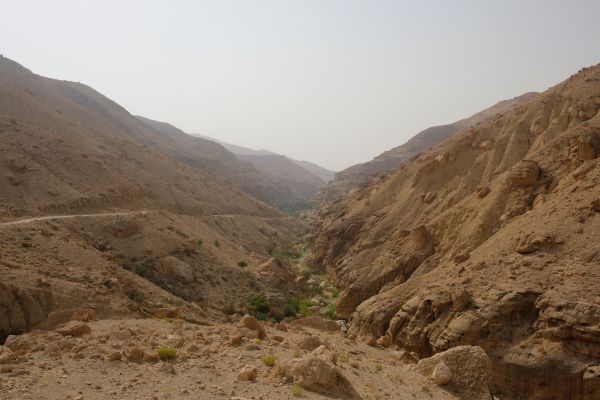The image captures a desolate canyon with light beige, sandy hills stretching obliquely on either side, giving the appearance that rainwater would naturally funnel down into the valley. The rugged landscape is dotted with large stones, scattered among smaller rocks, and the canyon floor is layered with patches of lush green plants, grass, and moss, concentrated in deep crevices. A small path can be seen winding along the base of the left-side mountain. The sky above—occupying about 20% of the photo in a distinct V-shape—is uniformly light gray, enhancing the stark, earth-toned scenery. The distant hills fade into an indistinct gray hue, reinforcing the arid and remote atmosphere of the canyon.